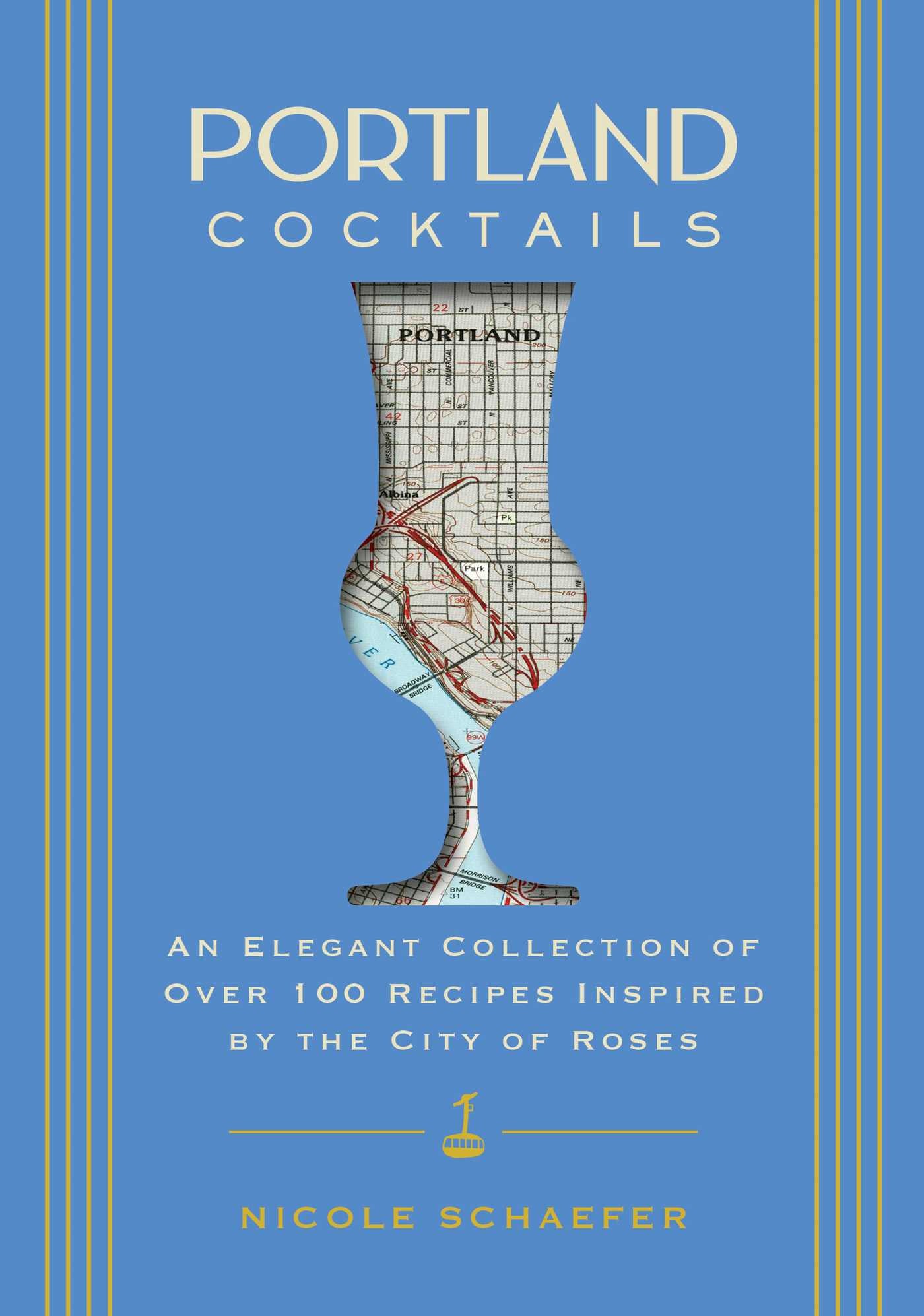The cover of the book features a light blue background with distinctive vertical stripes—four thin lines on each side, both left and right, in identical yellow. The book's title, "PORTLAND COCKTAILS," is prominently displayed at the top; "PORTLAND" is in a bold, all-caps font, while "COCKTAILS" appears in a smaller all-caps font. Centrally featured is an image of a cocktail glass, intricately filled with a map of Portland, showcasing its roadways, lines, and a bit of a river, resembling a grid. Beneath the glass image, the text reads in all capital letters, "An elegant collection of over 100 recipes inspired by the City of Roses." Below this phrase, there is an image of a yellow vehicle resembling a form of transportation. At the bottom, the author's name, "Nicole Schaefer," is displayed in yellow letters.